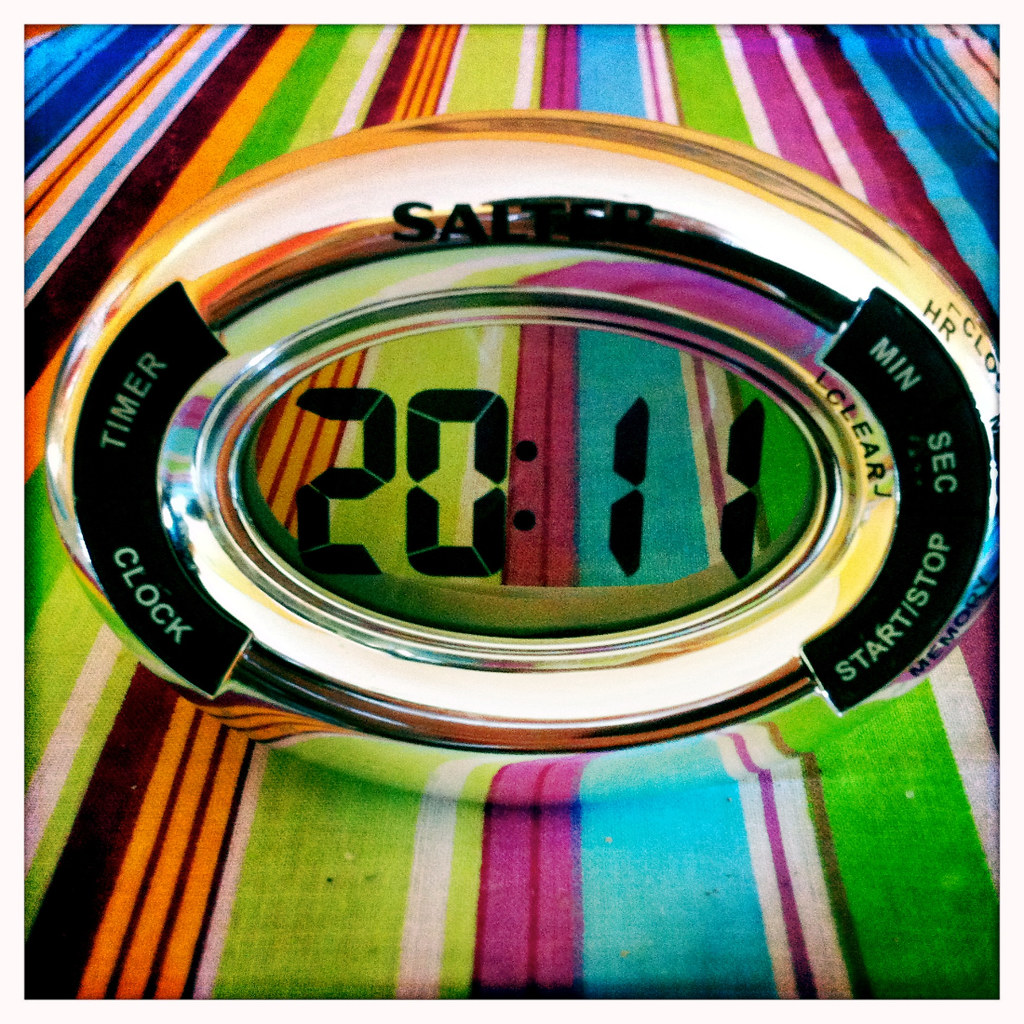The image showcases a digital clock lying on its side. The clock is oval-shaped with a golden metallic exterior, featuring a reflective oval mirror at its center. Black digital numbers display the time as 20:11. Surrounding the display are various functions labeled in white text, including "Clock," "Timer," "Minute," "Second," "Start," and "Stop," each housed within small black C-shaped segments.

The clock rests on a vibrant piece of fabric adorned with an array of colorful stripes. From left to right, the stripes include an array of colors: blue, orange, light blue, brown, orange, medium green, light green, white, brown, orange, lime green, white, purple, blue, white, green, white, purple, white, purple, brownish, light blue, dark blue, medium blue, and white. The multitude of colors in the fabric adds a lively and dynamic backdrop to the clock, creating a visually rich and engaging scene.